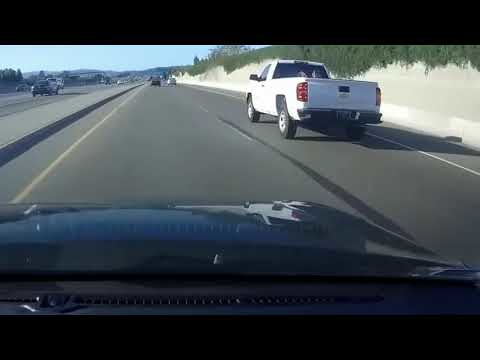This square color photograph, taken from inside a car or possibly a truck, captures a scene from a four-lane highway. The perspective is from the left-hand lane, looking down the road ahead. The front part of the interior is visible, highlighting the black dashboard and the black bonnet of the vehicle. A thin black stripe frames the photo across the top and bottom edges.

In the right-hand lane is a white pickup truck with black wheels and white rims. Ahead in the distance are two more cars traveling in the same direction. The opposite lanes are separated by a brownish median strip, with a car followed by another car visible against a backdrop of trees and hills or mountains. To the right side of the road, there is sand interspersed with green foliage, including large bushes and a single tree positioned in the top middle part of the frame. The road itself is marked by a yellow line on the left, white lines on the right, and white dotted lines down the center.